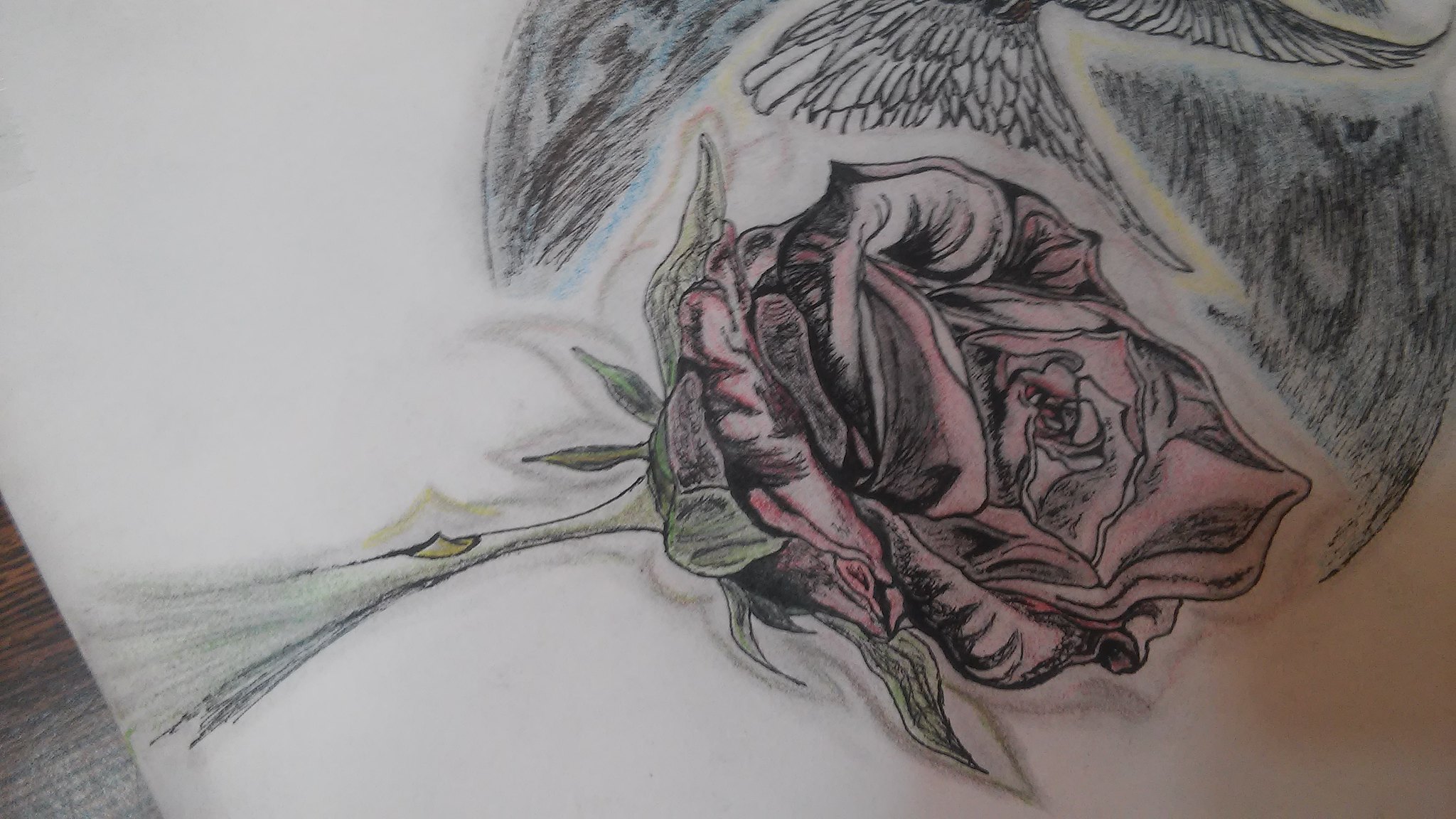This image depicts a detailed, colored pencil drawing on white paper, slightly angled up to the right, with a brown table visible in the lower left corner. The focus of the drawing is a large, red rose with intricately shaded petals, featuring darker tones for depth. Surrounding its base are green leaves with subtle shading. The rose's stem extends downward, displaying a prominent single thorn on the upper side. Above the rose, a bird appears to be mid-flight, its tail fanned out wide, with detailed markings for feathers, and partially visible wings shaded in dark black and white, extending towards different directions. The overall composition highlights the contrast between the vibrant red rose and the monochromatic elements of the bird and background, enriched with detailed shadowing to create a realistic effect.